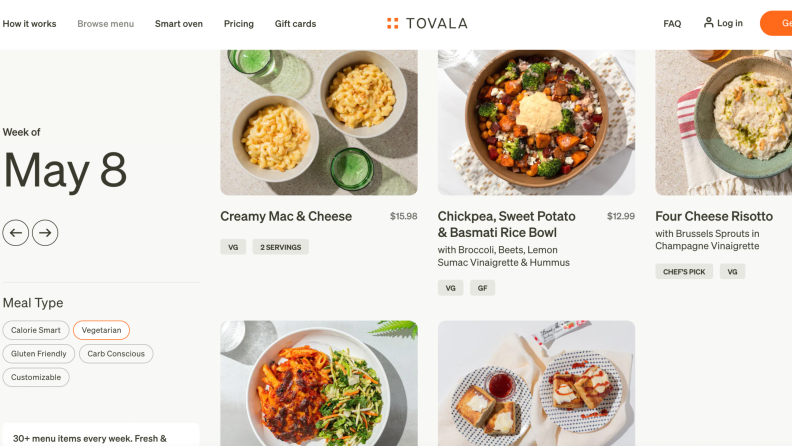This is a detailed screenshot of the Tovala webpage. At the very top navigation bar, the options include "How it works," "Browse menu," "Smart oven," "Pricing," "Gift cards," "FAQ," and "Login." Running vertically on the left side of the page are the categories for meal selection: "Week of May 8," "Meal Type," "Calorie Smart," "Vegetarian" (which is highlighted), "Gluten Friendly," "Carb Conscious," "Customizable," and a note stating there are "30+ Menu Items Every Week."

To the right, the page showcases several enticing menu items through photographs:
1. **Mac and Cheese:** Priced at $15.98 for two servings (VG). The image displays two white bowls filled with rich, orangish-yellow macaroni and cheese, accompanied by two pale green water glasses.
2. **Chickpea Sweet Potato and Basmati Rice Bowl:** Priced at $12.99, this dish includes broccoli, beets, lemon, sumac vinaigrette, and hummus (VG, GF). The visual shows a brown bowl brimming with the colorful rice bowl ingredients.
3. **Four Cheese Risotto with Brussels Sprouts and Champagne Vinaigrette:** This dish is marked as "Chef’s pick" (VG), although the price is cut off at the right edge. The presentation features a grayish-green stoneware bowl placed on a white fringed towel with red horizontal stripes at the top. The risotto appears creamy with a garnish of green herbs.
   
At the bottom of the screenshot, there are two partially visible images:
1. The left image shows a white bowl with a reddish-orange substance likely on the left, paired with a salad on the right.
2. The second image features what seems to be toast. The plates are white with small blue dots, with the toast on the left plate having a smear of butter on each piece and a small glass dish containing an unknown red substance. The plate on the right includes toast adorned with butter and red syrup or other similar substance.